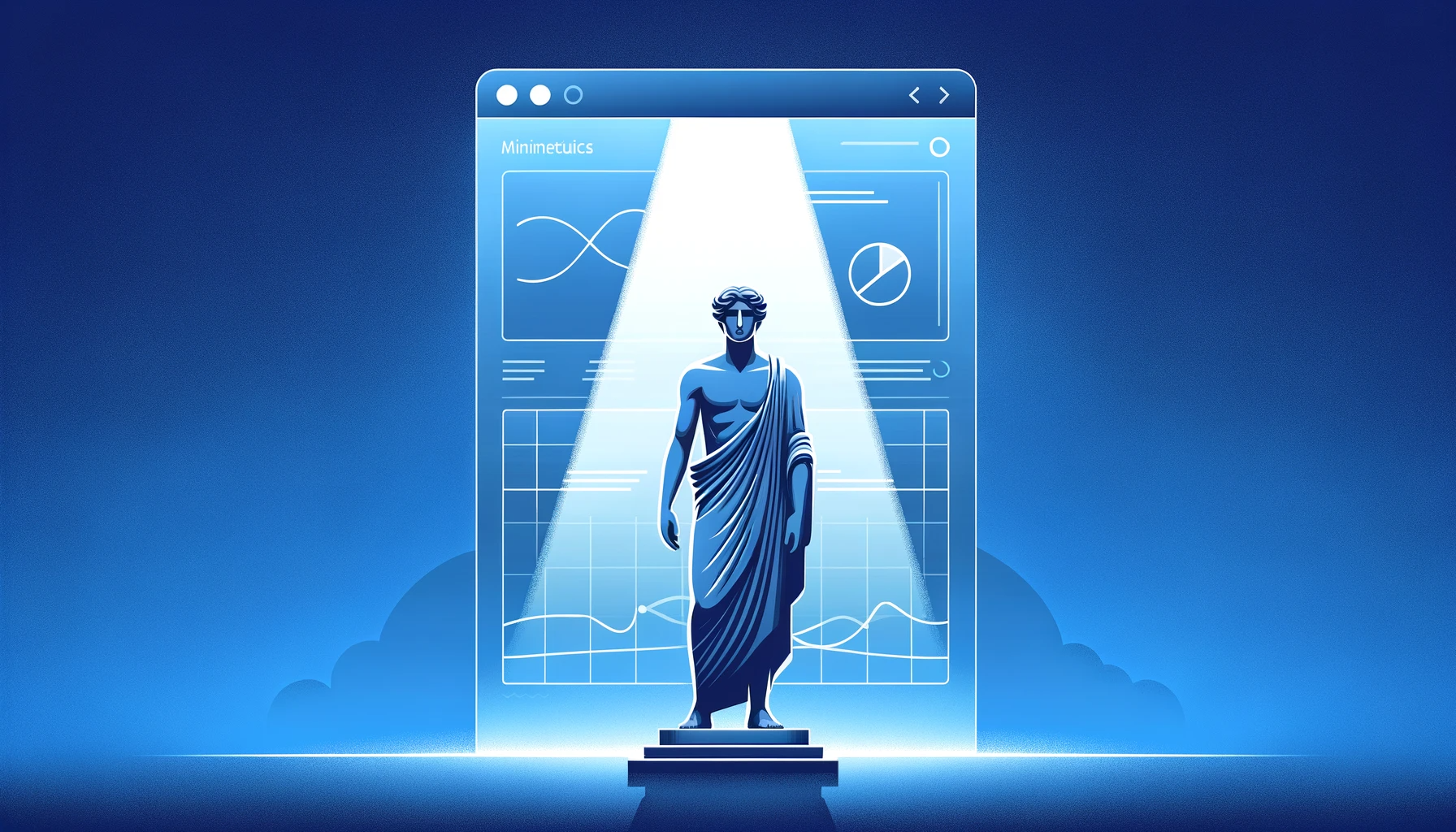The digitally created artwork features a horizontally rectangular image dominated by shades of blue and white, with no specific border. At the bottom center stands a majestic statue of a human male, depicted wearing a tunic draped over one shoulder, leaving his other shoulder and arm bare. His thick, curly hair and the detailed tunic accentuate his godly appearance. The statue stands on a three-step pedestal, which elevates him and adds to his grandeur. 

A spotlight from above illuminates the statue, casting a dramatic light that not only highlights his form but also radiates to the left and right from the base. Behind the statue is a representation of a digital interface, resembling a computer or smartphone screen filled with various types of graphs and charts, including a notable line graph, a pie chart with a highlighted slice, and an infinity symbol on the left. These digital elements add a modern contrast to the classical statue, all set against a solid blue background with a cloud-like silhouette.